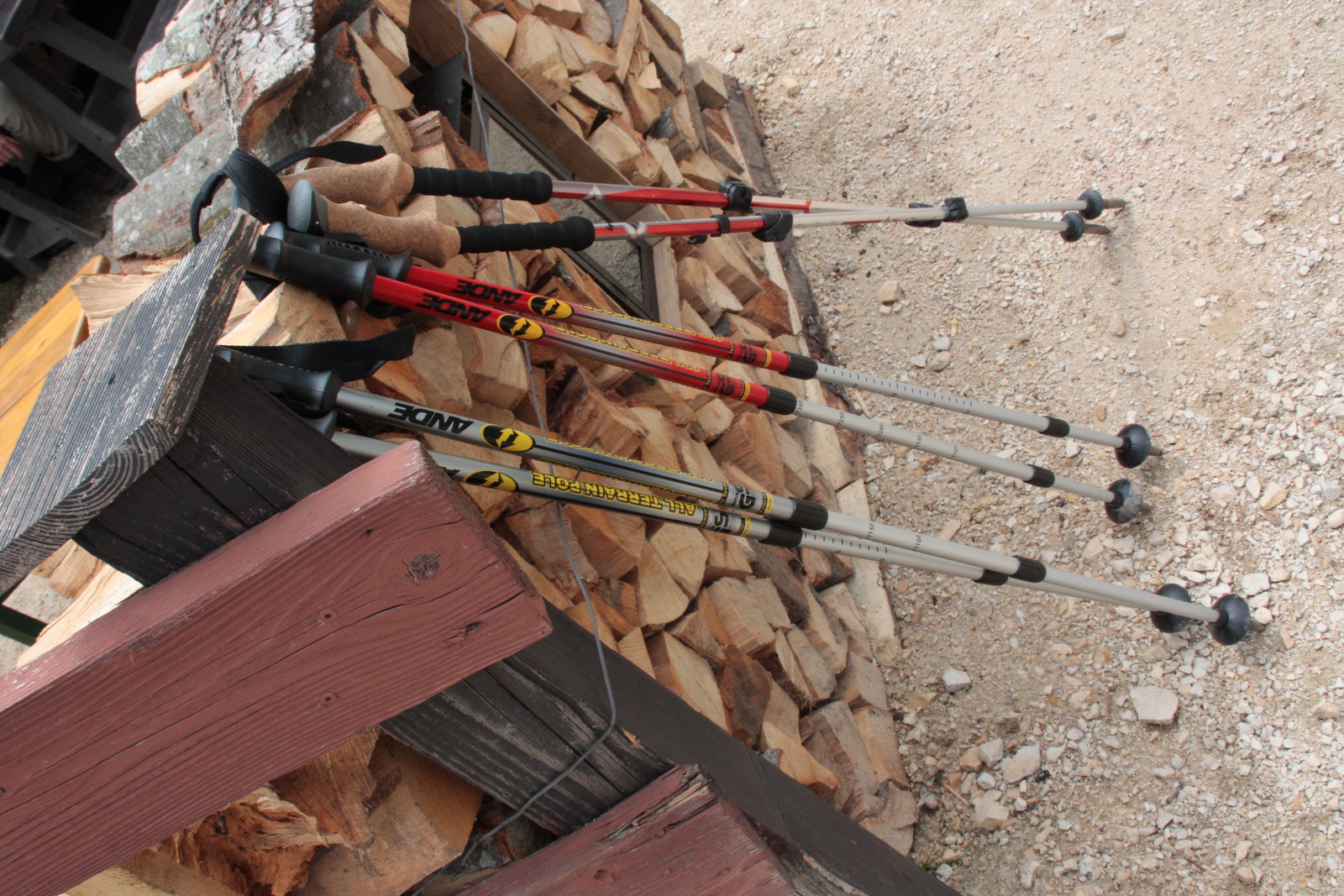The image captures an outdoor work area with a sideways view showcasing a makeshift wooden storage bin for logs and several hiking sticks propped against it. The ground is covered in a mix of gray and beige rocks and pebbles, creating a pale sandy-colored dirt surface. The storage bin is constructed from red and black wooden blocks forming a rectangular enclosure.

Within the storage, there's a variety of stacked wooden logs, featuring triangular and square shapes, and shades ranging from light brown to dark grayish brown. Leaning diagonally across the pile of firewood are six metal hiking sticks. These sticks vary in color: some are silver with black writing, while others are red with black writing and a yellow logo. All the sticks feature black handles at the top. The image captures the detailed textures of the outdoor setting, from the rugged terrain to the contrasting hues and materials of the logs and hiking equipment.